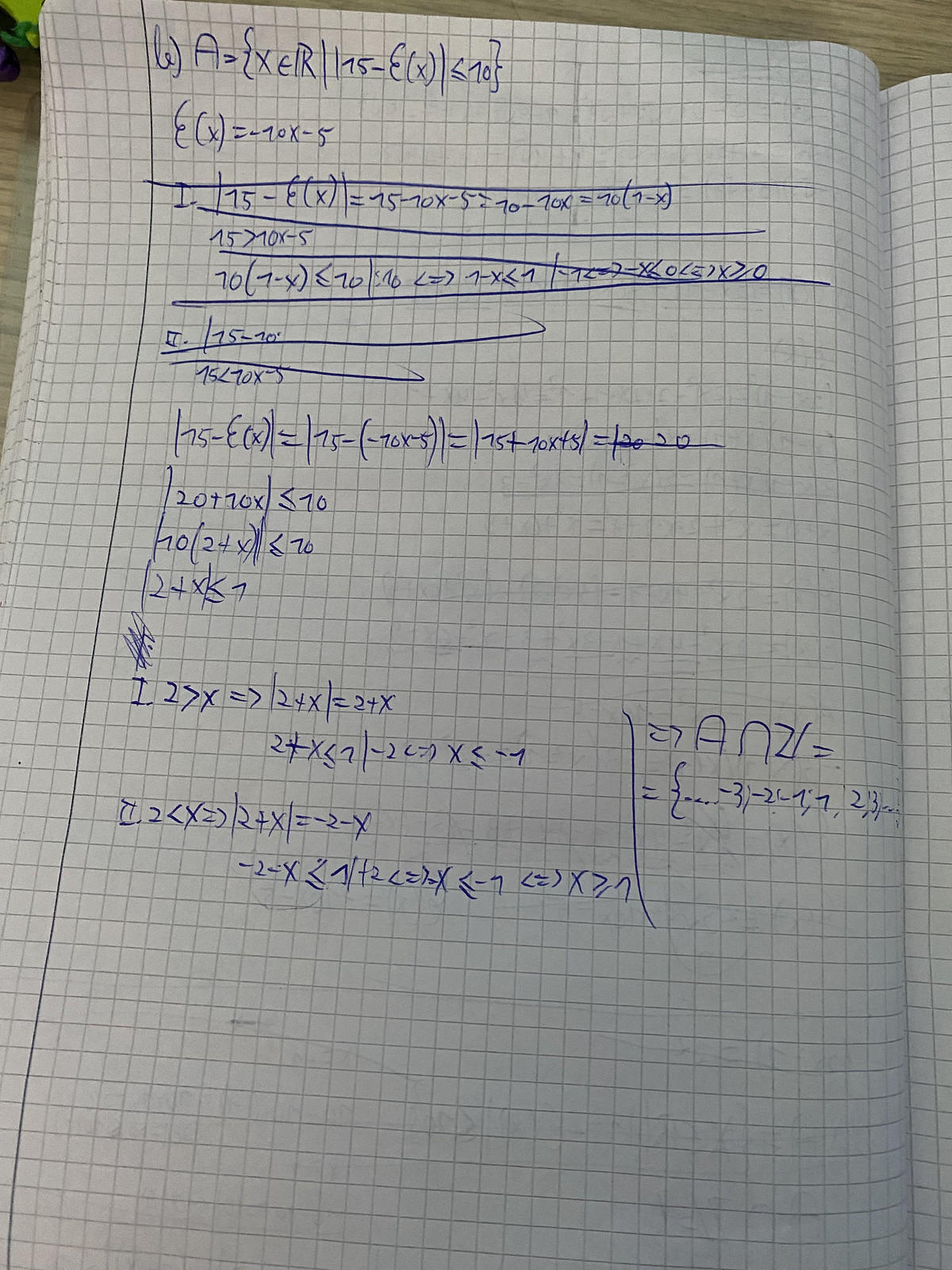The image depicts a large sheet of graph paper, likely from a notebook slightly larger than the standard 8.5 x 11 inches. The paper has light blue squares characteristic of graph paper, and it's filled with handwritten algebraic problems and calculations. The work begins with the equation \( \epsilon x = -70x - 5 \). There are two initial attempts to solve the problem, marked by Roman numerals I and II, but these efforts are crossed out entirely.

Further down the page, a second set of calculations appears, extending across the page as the person continues to work through the algebraic problem. Near the bottom right corner, the phrase "ANZI =" is written, followed by a bracket containing a sequence of numbers: -3, -2, -7, 7, 2, 3.  

Finally, the page culminates in another pair of attempts marked by Roman numerals I and II, where it seems the person believes they have arrived at the correct solution to the equation. The detailed and methodical approach, despite the corrections and numerous calculations, illustrates a determined effort to solve the algebraic problem.